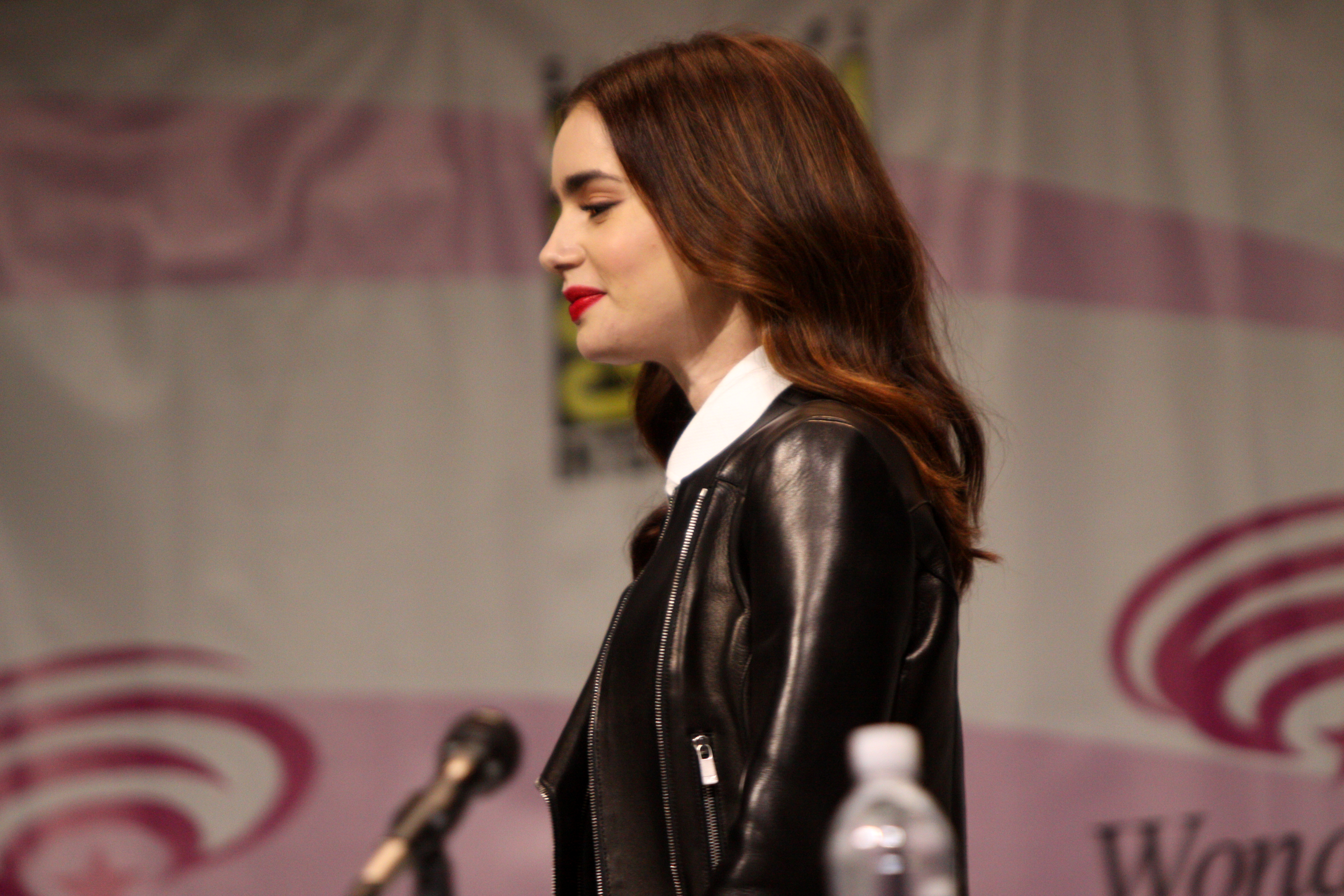The photograph captures a young actress with strikingly thick black eyebrows, a pointed nose, and wavy brown hair tinged with red at the tips. She is adorned with bright red lipstick that stands out against her pale white skin. Clad in a black leather jacket featuring zipper pockets and a black shirt with a white collar, she exudes a confident and stylish appearance. The image appears to be taken at Comic-Con, evidenced by the prominent yellow Comic-Con sign in the background. She seems to be on stage, possibly participating in a panel, as suggested by the microphone and bottle of water positioned in front of her. The subtle details in the background, including swirling patterns on the curtain, add to the dynamic setting. The partial text "WOND" suggests a possible connection to the Wonder Woman franchise, hinting at her role in a superhero movie. The actress, looking to the left, is the focal point of the photograph.